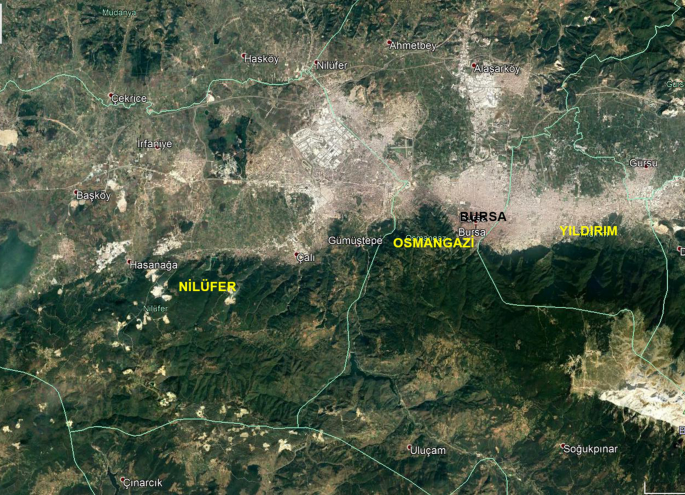The image, likely a satellite view from Google Maps, features a landscape seen from a completely top-down perspective. Light bluish-green lines crisscross the image, suggesting they are dividing lines rather than natural rivers. In the image, the bottom half is predominantly green, depicting a more mountainous region with moderate elevation, whereas the top half is characterized by lighter colors, such as white, gray, and beige, indicating possible settlements like towns or villages.

In the center-left of the image, the word "Nilufer" appears in yellow, while "Osman Gazi" is positioned centrally and "Ilyirlim" is on the right-center, both in yellow as well. Near the word "Osman Gazi," "Bursa" is marked in black towards the right side of the image. Additionally, there is a small water body located towards the left side. Various places are labeled in different colors, with the text in white, yellow, and black, all appearing to be in a language that is not immediately recognizable.